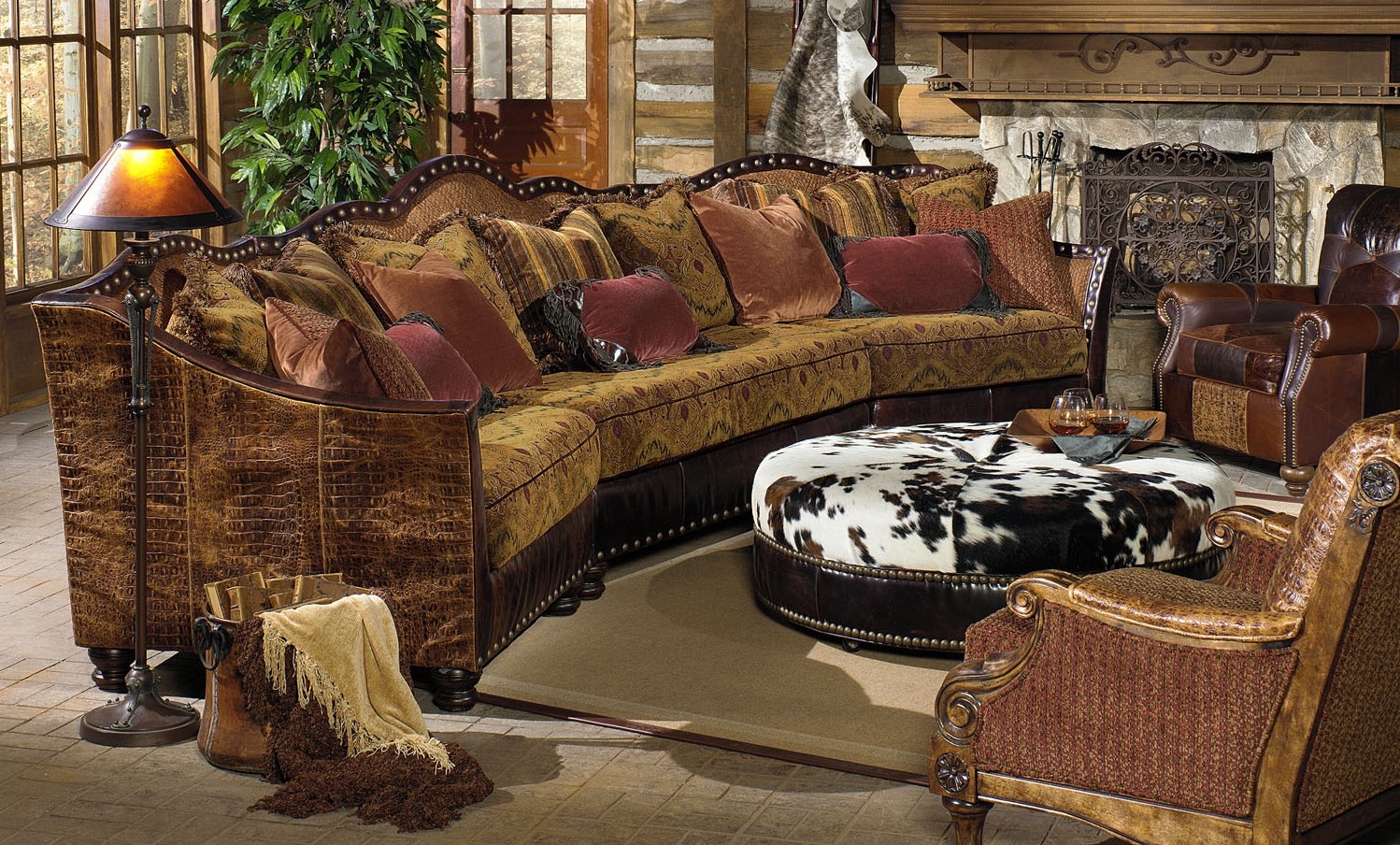The image showcases a beautifully detailed living room with a somewhat elaborate design. Dominating the space is a large curved sofa, capable of seating around six people, featuring a brown and orangey hue adorned with numerous red pillows. This sofa curves around a circular, black and white cowhide ottoman that serves as a central piece, with a tray holding three glasses of wine resting atop it. To the right of the sofa, two comfortable, brown leather chairs with hand rests and cushions are positioned, enhancing the room's cozy ambiance.

The space is illuminated by a black lamp with an orange top, complemented by additional brown-colored lighting. A brown rug lies on the beige floor, providing warmth and texture. The left side of the room is lined with large windows and a door, offering a view of the outside foliage and allowing natural light to flood in. A green plant is placed by these windows, adding a touch of nature indoors.

In the middle of the room, a fireplace with an elaborate stone design and a metal grate becomes a focal point, featuring an intricate shelf above it. Horizontal wooden slats adorn the surrounding walls, adding rustic charm. Additionally, near the couch on the left side, there is a basket with a white blanket draped over it, contributing to the inviting and lived-in feel of the room.